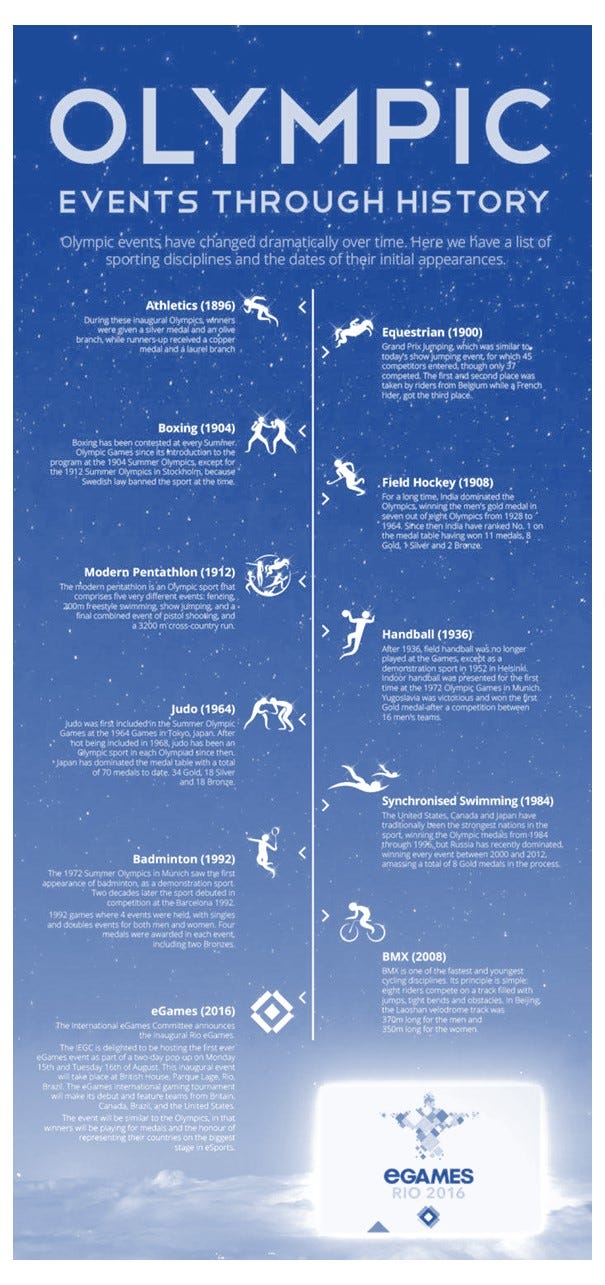This is a detailed graphic image depicting the evolution of Olympic events through history, arranged in a vertical timeline. The background transitions from dark blue to almost white, adorned with stars and clouds as it moves downward. The title at the top center reads "Olympic Events Through History" in prominent white text. Below the title, there is a chronological list of sporting disciplines and the dates of their initial appearances, positioned alongside their respective icons, which include athletes boxing, wrestling, playing badminton, and cycling.

A white line runs down the center of the image, dividing the events listed on the left and right sides. Athletically themed icons and text for each event include: Athletics (1896), Equestrian (1900), Boxing (1904), Field Hockey (1908), Modern Pentathlon (1912), Handball (1936), Judo (1964), Synchronised Swimming (1984), Badminton (1992), BMX (2008), and E-Games (2016).

At the bottom right of the image, a bright beam of light highlights the logo for "eGames Rio 2016," featuring an illustration of the iconic Christ the Redeemer statue from Rio de Janeiro. Beneath each event header, small white text provides additional details. The overall design is visually striking with its gradient background, neatly organized timeline, and comprehensive blend of text and imagery.